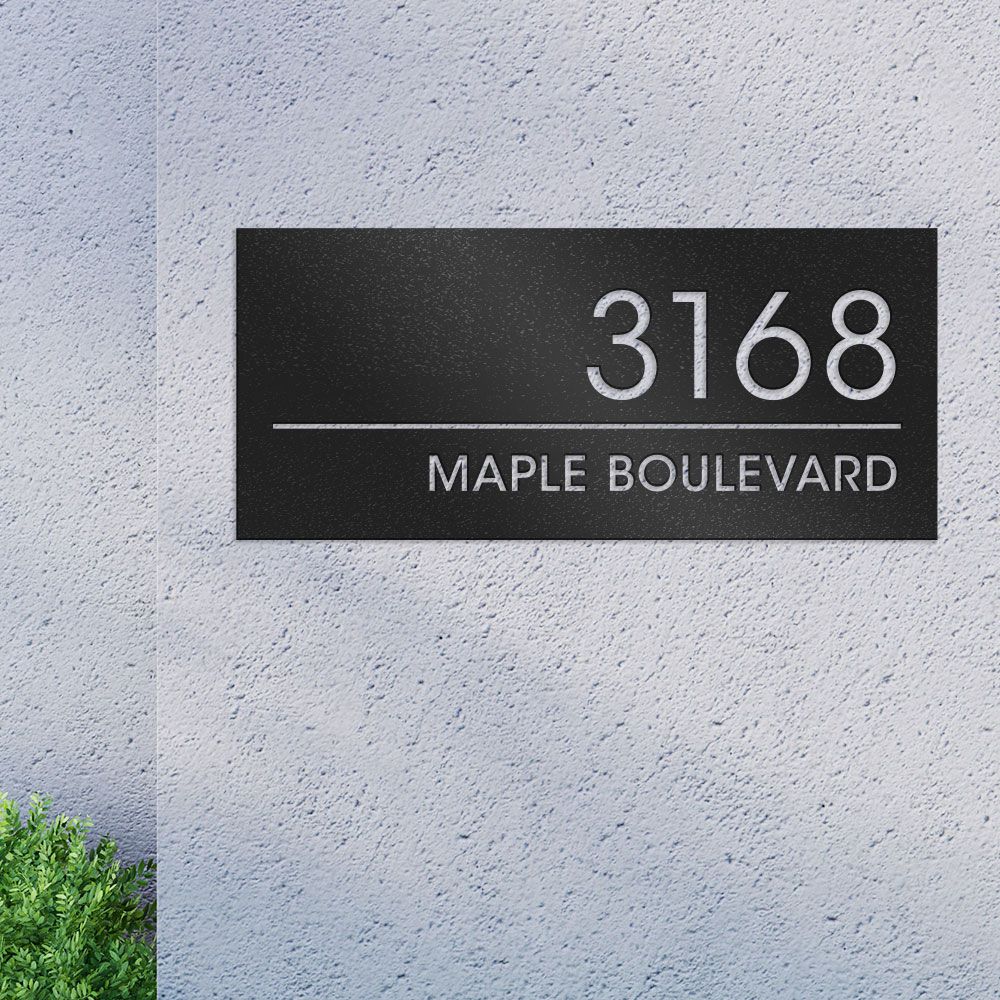The image displays a close-up of a light gray, textured stucco wall with a professional black plaque serving as an address marker. The plaque, positioned towards the upper half of the wall, prominently features the white-engraved numbers "3168" with "Maple Boulevard" written below, separated by a horizontal line. The scene is picturesque, well-lit, and likely captured during a sunny day, evidenced by the slight shadows cast on the wall. Small green shrubs are visible at the bottom and left corner of the photo, extending slightly up the wall. The background is black, further highlighting the wall and plaque. The photograph may be intended for advertisements or directional purposes, showcasing the building's address in a clear, visually appealing manner.